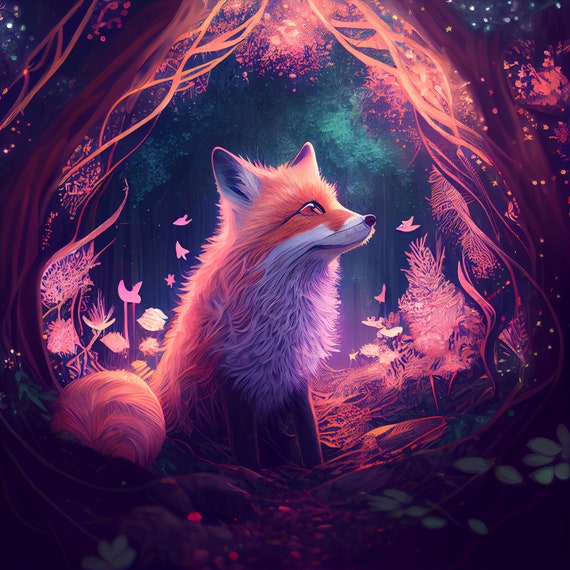Digital artwork depicting a serene scene featuring a red fox as its centerpiece. The fox, characterized by its rich red fur, white chest, and white muzzle, sits gracefully facing to the right. Its brownish eyes and a small brown nose add to its lifelike charm. Notably, its plush, fluffy tail is curled around its body, extending towards the front of the image.

Surrounding the fox is an enchanting, mystical forest, with textured, purplish trees rising on either side. These trees frame the fox and contribute to the image's fairy-tale atmosphere. In the background, smaller trees with light pink foliage and intricate textures add depth to the scene. Further back, some birds are visible, flying above the dense forest.

Towards the lower part of the image, the forest appears darker and more mysterious, transitioning to a greenish tint at the top, reminiscent of tree canopies. The top edges of the artwork hint at a sky adorned with subtle stars, enhancing the magical feel of the scene. The dominant color palette of purples and pinks is complemented by touches of green from what appears to be leaves or moss sprouting on the forest floor.

Overall, the image possesses a dreamy, ethereal quality that captures the viewer's imagination and transports them into a captivating woodland realm.